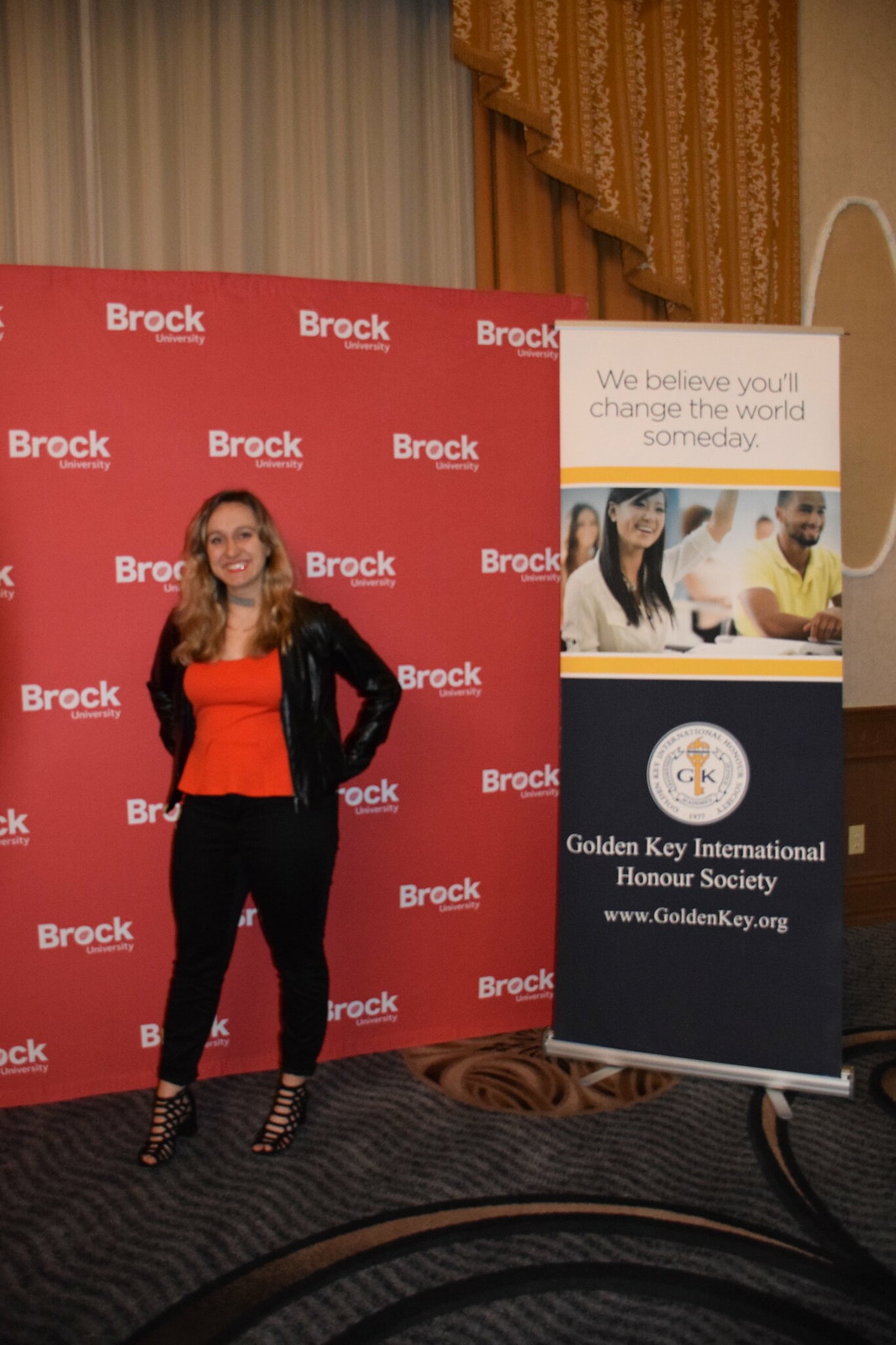In this photo, a young woman with dirty blonde, straight hair is posing in front of two promotional displays. She is dressed in a sleek black leather jacket over an orange top, paired with tight black dress pants and stiletto heels. She accessorizes her look with a gold necklace and a tattoo on her neck. One of the displays behind her is a large, red wall with "Brock University" prominently featured. The other display reads, "We believe you'll change the world someday," and includes the logo for the Golden Key International Honor Society (www.goldenkey.org). This display also features an image of students, including a woman raising her hand and a dark-skinned man sitting beside her. The setting appears to be a conference room or a stage within Brock University's premises, likely for an award ceremony or an open house event.